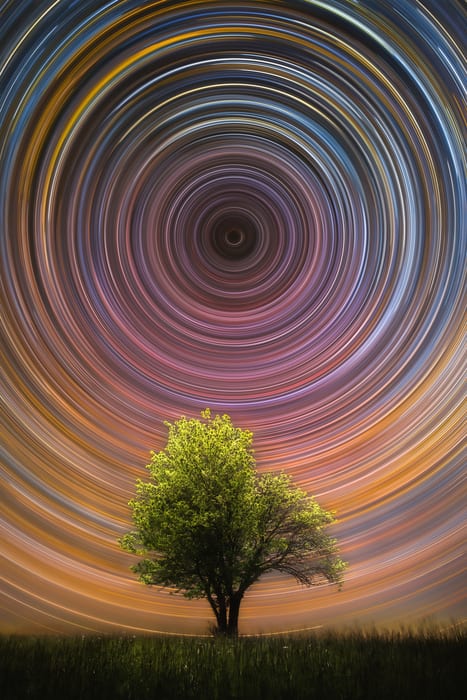The digital art poster presents a vivid and surreal scene featuring a solitary tree with bright green leaves and dark brown branches, standing on a silhouette-like ground covered with dark green grass. The most striking element is the sky, which is depicted as a mesmerizing spiral of colors. Starting from a deep purple at the center, the spiral expands outward through gradients of blue, yellow, orange, and pink, creating an entrancing and dynamic backdrop. The swirling sky and the lit treetop suggest a time-elapsed effect, capturing the essence of stellar movement and cosmic light trails. This captivating piece appears designed to be a framed art print, ready to adorn any wall with its enchanting and otherworldly beauty.